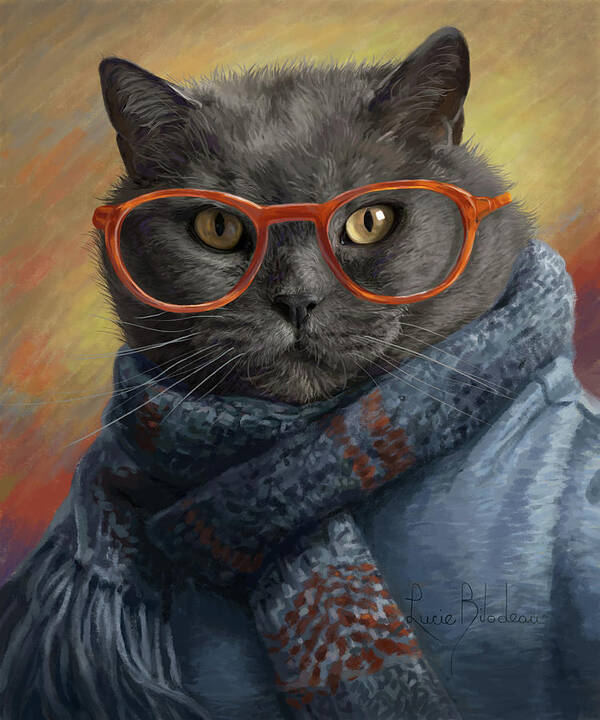This visually engaging digital artwork depicts a dark gray cat with piercing yellow eyes, each featuring vertical pupils, creating an intense gaze straight at the viewer. The cat also sports a distinctive pair of red-framed (or possibly orange) glasses, adding an unexpected, whimsical flair. Its attire includes a striking blue scarf with subtle brown and orange enhancements and tassels hanging off to one side, wrapped warmly around its neck. Complementing the scarf is a blue shirt, contributing to the cat's anthropomorphic charm. The background is an abstract, colorful blend of swatches including yellow, blue, brown, and red, creating a vibrant, chaotic backdrop that brings focus to the cat. The artist's signature, identified as Lucie Belladio, is subtly placed in the lower right-hand corner, somewhat faint but present.